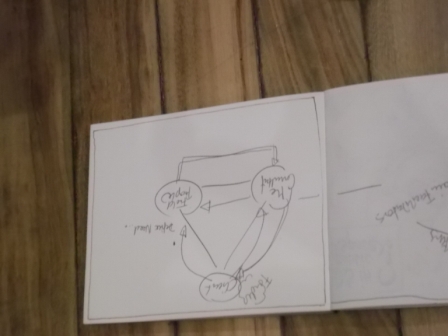A rectangular photograph captures an open booklet at its center, with the top and bottom sides of the image being longer than the left and right sides. The booklet, oriented upside down, reveals two of its blank, rectangular-shaped pages. The right page is partially cropped out of the frame. Written in pencil, the notes are oriented towards the bottom edge of the photograph, rendering the text inverted. On the left page, the only legible word, "fabulators," is visible, accompanied by a line extending to the adjoining page. The adjacent right page features a thin pencil-drawn square framing its perimeter. Inside this square sits a pentagon, adorned with three circles and arrows pointing between them. Although multiple lines of cursive text are present, they are blurred and difficult to decipher.